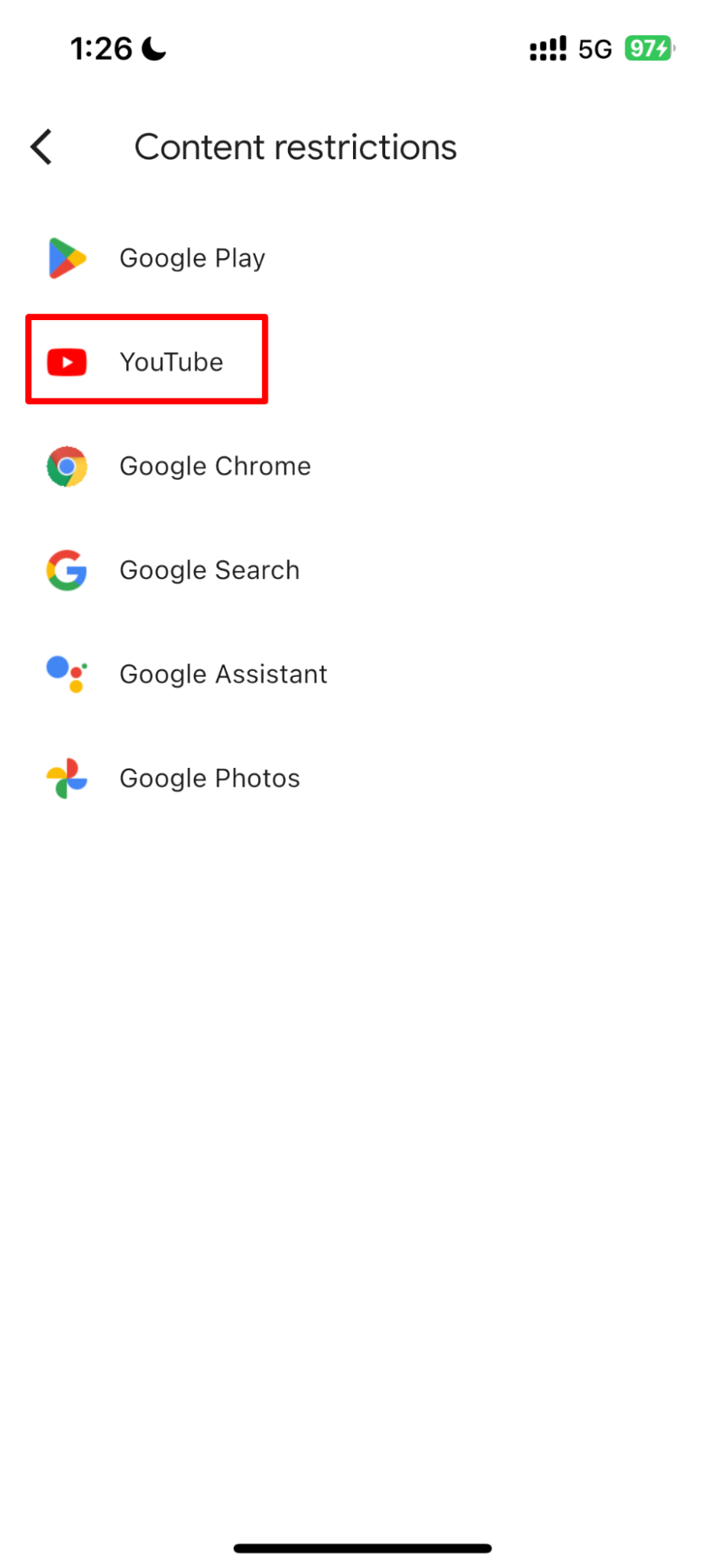This detailed caption tells the full story of an image captured from a phone screen, highlighting various content restriction settings. 

"A late-night screenshot taken at 1:26 a.m., evident from the moon icon next to the time, reveals a fully detailed interface of content restriction settings on a smartphone. The phone was connected to a 5G network with full signal strength and was charging, as indicated by the green battery icon showing 97% power. The interface displays a white background with black text for optimal readability. In the top-left corner is a back arrow labeled 'Content Restrictions', suggesting the navigation to this specific settings page. Central to the screenshot is a list of applications and programs available for restriction. At the top of the list is 'Google Play', followed by a highlighted 'YouTube' indicated by a red selection box. Subsequent entries include 'Google Chrome', 'Google Search', 'Google Assistant', and 'Google Photos'. This image captures a user customizing or reviewing content restriction settings for various Google applications on their device."